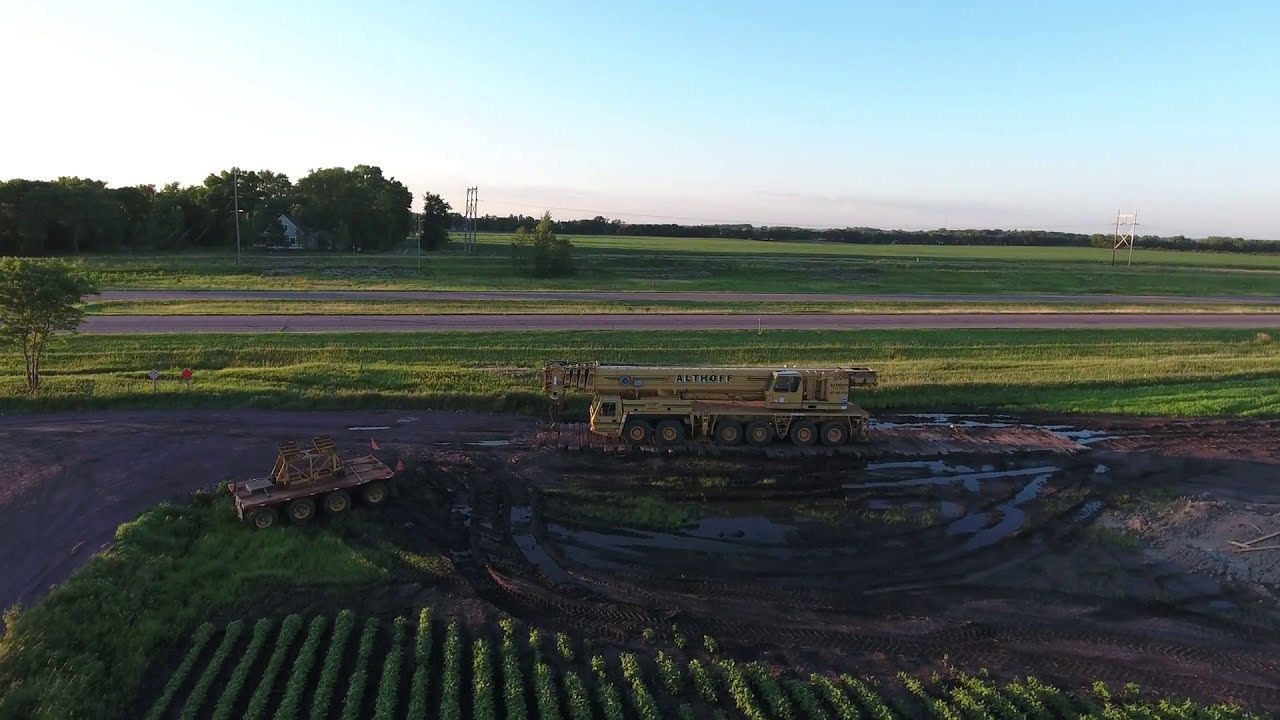In this detailed drone-captured color photograph, a scenic rural farming area is laid out in a landscape orientation, showcasing both agricultural and mechanical elements with stark clarity. At the bottom of the frame, meticulously planted rows of crops, possibly shrub-like, run vertically, their neat arrangement highlighted by the soft light of the setting sun. Central to the image is a large, light yellow farm tractor, identifiable by its six visible tires and a crane-like hook on top. The tractor's bulk has created deep treads in the muddy terrain it occupies, suggesting recent activity, perhaps due to watering operations or rain. Inscribed with the name "Althoff," this prominent piece of equipment stands out against the varied textures of the farmland. To its left is a smaller, orangish-red tractor, less imposing but contributive to the scene’s narrative. Beyond these machines, a small paved strip hints at a road or simple highway, bifurcating the scene and leading into a verdant pasture. The harvested section of the pasture, dirt trails, and a dense stand of dark green trees at the top left adds depth and contrast, all under a light blue sky that casts a serene hue over this representational depiction of rural life.